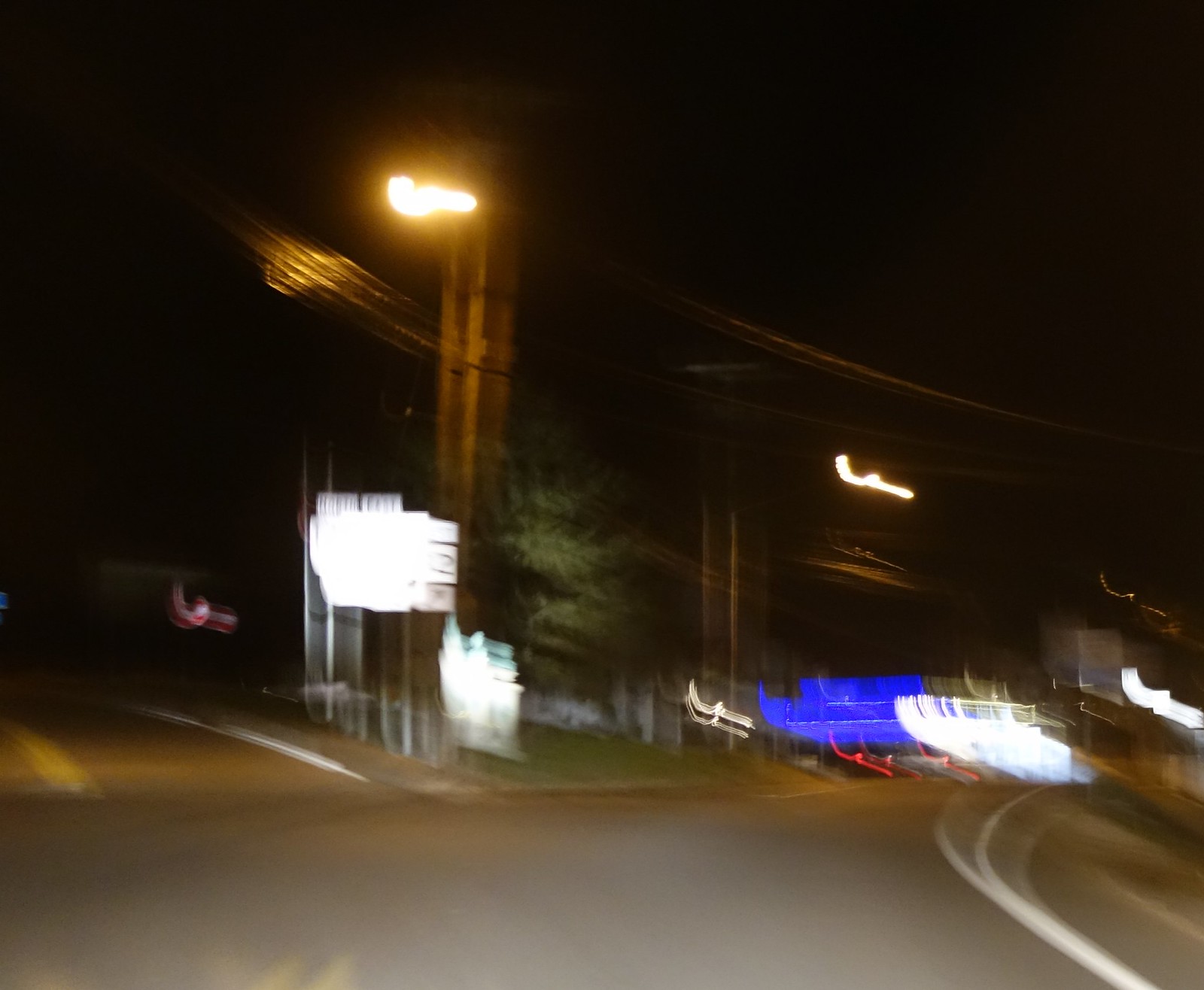The image depicts a nighttime scene captured from a moving vehicle, resulting in a very blurry photograph. The sky is pitch black, creating a stark backdrop against the various blurred lights. There's a prominent tall and bright, yet also blurry, streetlight illuminating the area. The scene appears to be an intersection with grey cement and winding roads adorned with white and yellow lines. Electrical poles and lines can be vaguely discerned, adding to the urban setting. Scattered throughout the image are blobs of blue, white, and red light, possibly reflections off vehicles or buildings. The road markings include solid white lines on the side and yellow lines down the center, indicating a fork where the road splits to the left and right. Additionally, there are white blurry blobs that might be street signs, one of which has a discernible number two. In the bottom right corner, a white squiggly line stands out in the darkness above a blue blur, adding to the sense of motion and confusion in the overall blurry night scene.